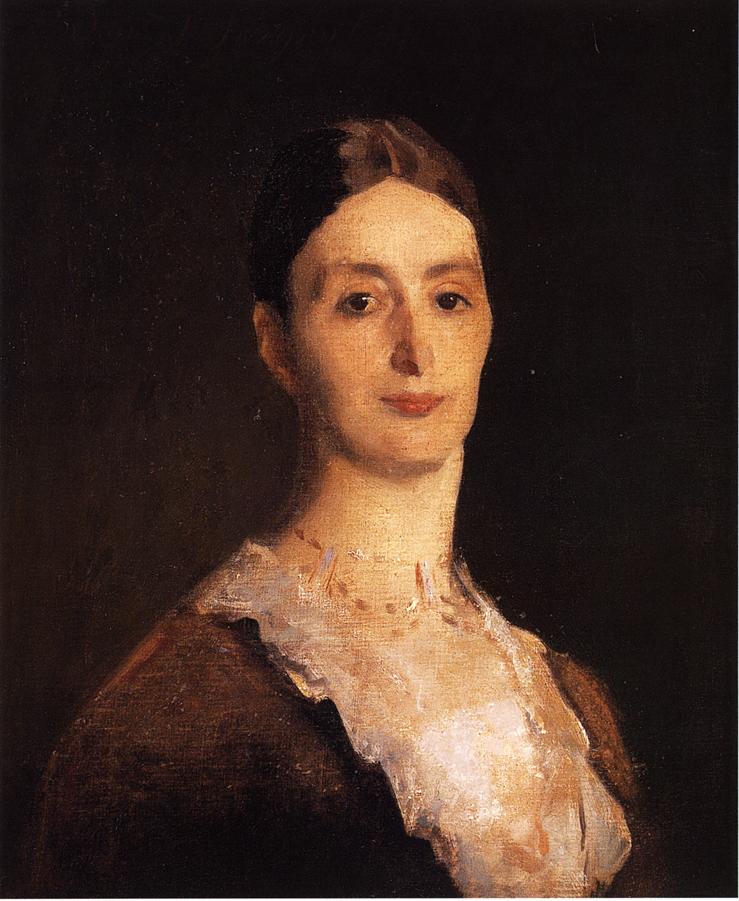This is a detailed portrait painting of a woman set against a dark brown or black background. The woman, who has tanned skin and dark brown hair that is slicked back and possibly tied into a bun, gazes directly ahead with a serious and stern expression, although there is a hint of a slight smirk or smile. Her hair is parted in the middle and pulled back behind her ears. She has thin, light brown eyebrows, droopy brown eyes, and a very thin, pointed nose. Her lips are pale red and closed, complementing her narrow, long face. 

The woman is dressed in a Victorian-style brown dress adorned with white ruffles around the collar area, with a white blouse visible beneath. Her attire includes a painted necklace, possibly beaded, with details that are faintly discernible, adding to the elegant yet austere look. The portrait captures her down to the shoulders, emphasizing her long neck and drooping shoulders. The overall tonality of the painting is predominantly brown, accentuating the starkness and somber mood of the portrait, which is intricately detailed and well-executed.